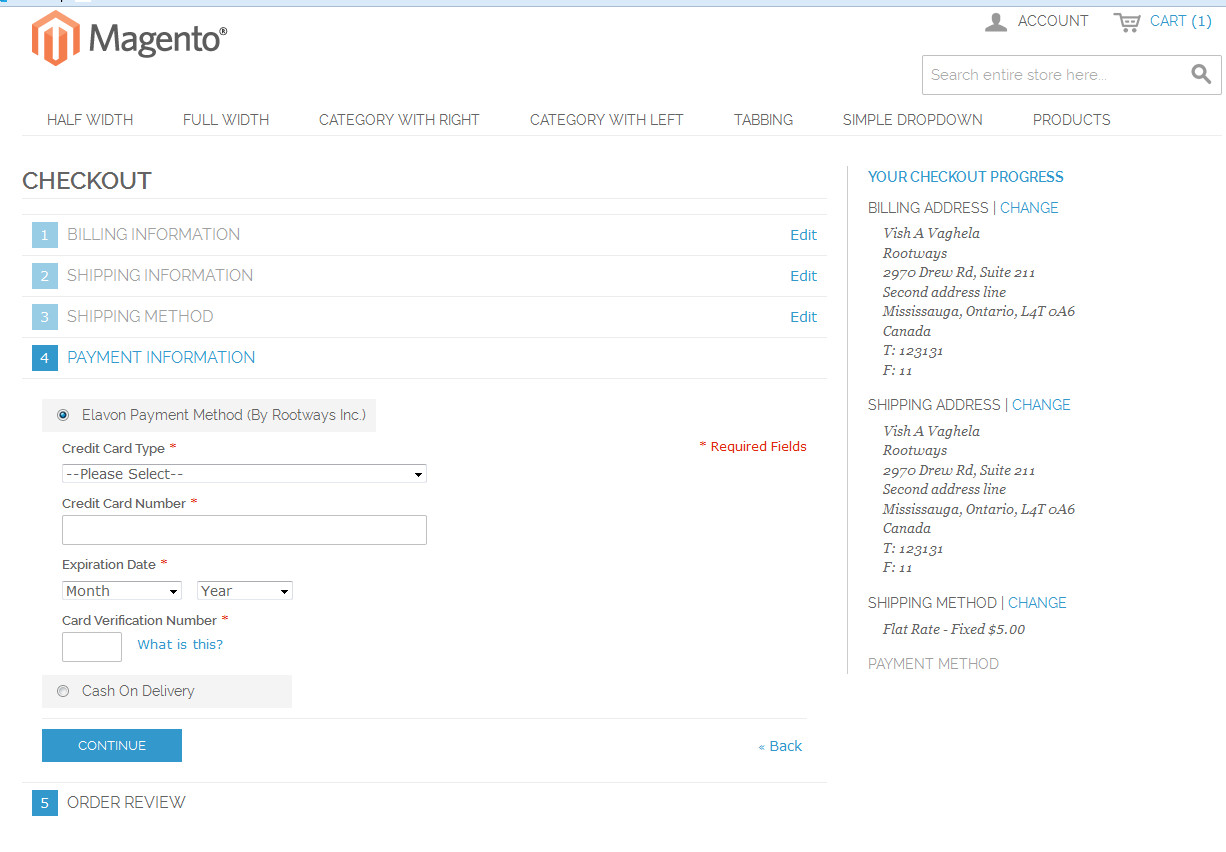The image depicts the checkout screen of the Magento company website. Prominently, the top left corner features an orange logo followed by the name "Magento," marked as a registered trademark. In the top right corner, icons for account login and a shopping cart are displayed, with the cart indicating it contains one item within blue brackets.

Beneath the header, a series of navigational headings spans the width of the screen, accompanied by a search bar on the far right. The headings listed include "Half Width," "Full Width," "Category with Right," "Category with Left," "Tabbing," "Simple Drop Down," and "Products."

Currently displayed is the checkout screen, structured around a series of sequential, numbered sections: 
1. Billing Information
2. Shipping Information
3. Shipping Method
4. Payment Information

The "Payment Information" section is highlighted in bold blue text, signaling the active step in the checkout process. Each of the preceding sections features a small "Edit" button on the right side, allowing users to make changes if necessary.

Within the "Payment Information" box, users are prompted to enter their payment details. Fields are provided for specifying the credit card type, entering the credit card number, expiration date, year, and card verification number. 

At the bottom of this section, a blue "Continue" button is prominently displayed, ready for users to proceed with their transaction.